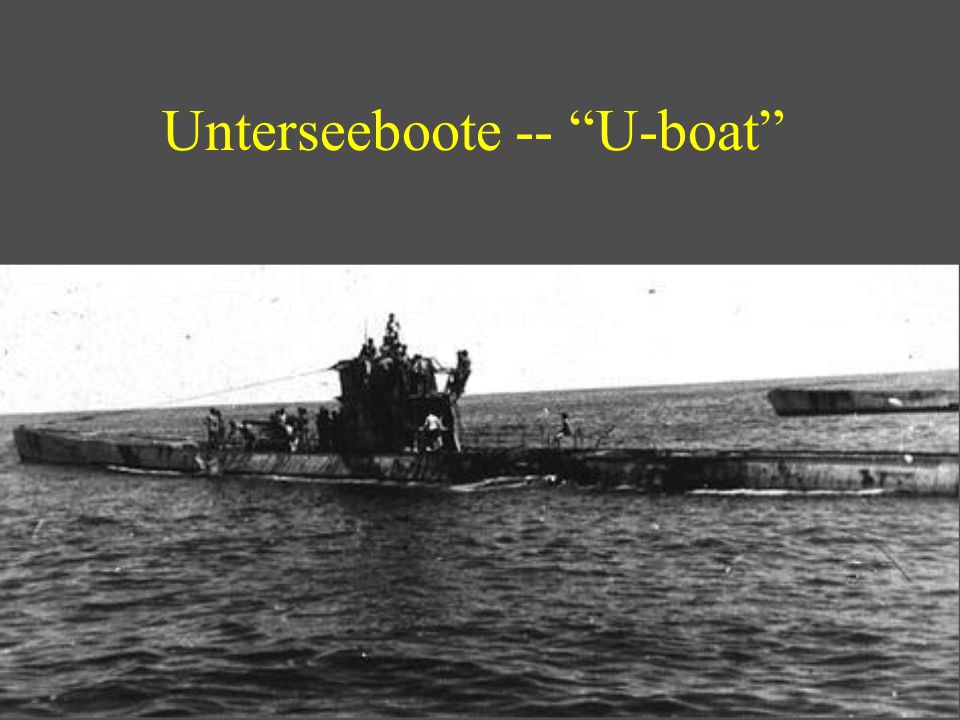This is a black and white photograph of a large, rusty U-boat, also known as an Unterseeboot (spelled U-N-T-E-R-S-E-E-B-O-O-T-E), floating in the middle of a calm ocean with slight choppiness and no significant waves. The image includes a gray border at the top with the word "UNTERSEABOOT" in bright yellow text, and the phrase "U-BOAT" in quotation marks. The submarine, which is elongated and narrow, appears somewhat weathered with dark patches that give it a dirty and unclean look. Several men on the deck are engaged in an activity involving a rope that extends into the water, possibly anchoring the boat or conducting some other task. In the background, another boat is faintly visible against the predominantly white sky.